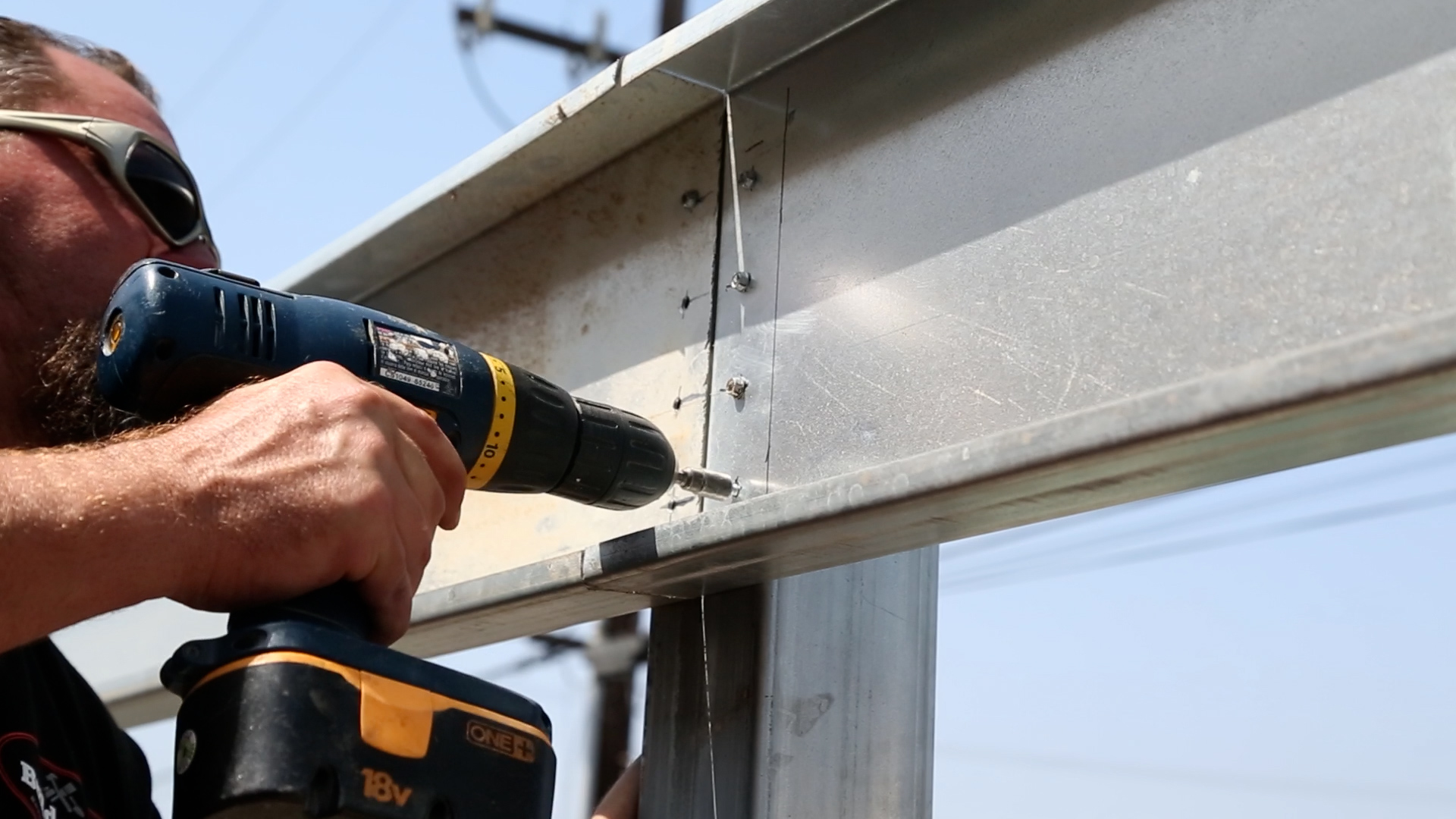A man with short, dark hair streaked with gray and a receding hairline is pictured on the left side of the photo, working diligently outdoors under a clear blue sky. He is using a power electric screwdriver or drill, which features a black front, yellow highlights, and a dark blue body, with the battery pack in black and yellow and marked "18V" in yellow letters. His hand, visible with some arm hair, grips the drill firmly at about chest level as he screws the fourth of eight screws into a steel beam. The man, who also has a blonde beard, wears Oakley-style gray and black sunglasses and a black shirt with a logo. Behind him, electrical lines and a light fixture are visible, adding to the industrious atmosphere of the scene.